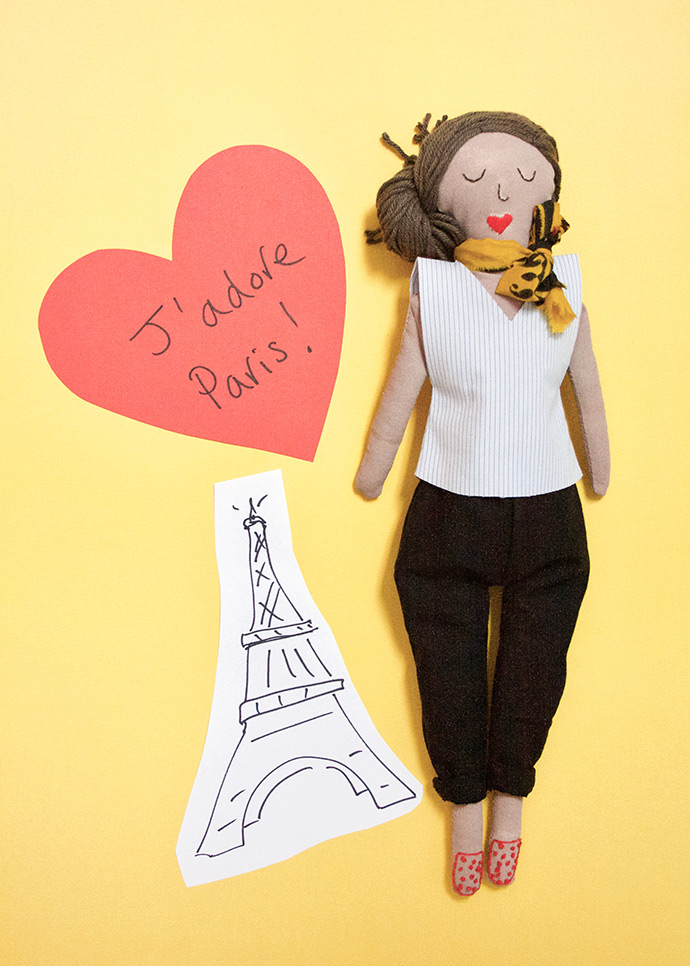The photograph features a horizontally aligned yellow background that showcases a heartfelt artistic expression of love for Paris. On the upper left side of the image, there's a prominent off-pink, misshapen heart, likely crafted from paper. The heart is slightly elongated and tilted to the left. Inscribed on this heart in a black pen is the phrase "J'adore Paris!" in a handwriting style, complete with an exclamation mark.

Beneath the heart, a roughly triangular piece of white paper carries a minimalist, sketch-like drawing of the Eiffel Tower, also done in black pen, echoing a Picasso-esque simplicity. To the right of these elements lies a handmade felt doll of a woman, extending almost the entire height of the photograph. 

The doll is fashioned from tan felt and features brown yarn hair pulled into an ornate bun on the left side of her head. Her eyes are just two little black U-shapes, giving the impression that they are closed, and she has red lips formed from a heart-shaped piece of felt. The woman wears a short-sleeve, vertically ribbed white shirt with a V-neck, black cuffed pants, and pink-pointed shoes with tiny white patterns. Between her pants and shoes, her felt skin is visible. Around her neck, she sports a yellow and black decorative scarf tied in a bow.

This detailed arrangement presents a charming, handcrafted homage to Paris, blending art, text, and a unique felt doll into a cohesive, visually stimulating composition.